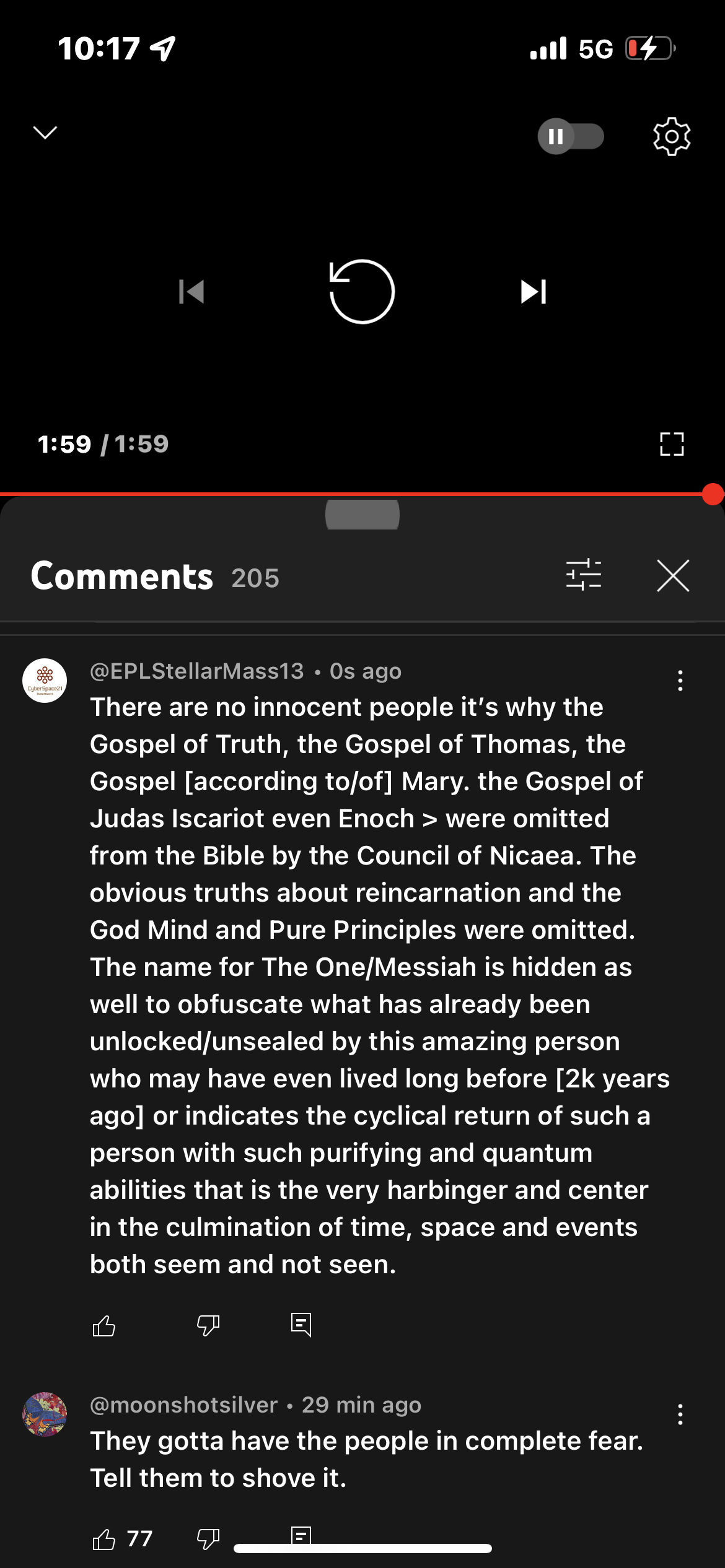This screenshot captures several elements from a user's YouTube app interface. At the top, it displays the current time as 10:17, indicates a full 5G signal, and shows the battery level as low but currently charging. The focal point of the screenshot is a YouTube video that just ended. The video is 1 minute and 59 seconds long and is from a user named @EPL_stellar_mass_13.

The top comment on the video, posted zero seconds ago by @EPL_stellar_mass_13, reads:

"There are no innocent people. It's why the gospel of truth and the gospel of Thomas, the gospel according to and of Mary, the gospel of Judas Iscariot, and even certain Gnostic texts were omitted from the Bible by the Council of Nicaea. The obvious truths about reincarnation and the God Mind and pure principles were omitted. The name for the one/Messiah is hidden as well to obfuscate what has already been unlocked/unsealed by this amazing person who may have even lived long before 2,000 years ago, or indicates the cyclical return of such a person with such purifying and quantum abilities that is the very harbinger and center in the accumulation of time, space, and events both seen and unseen."

Beneath this comment, another user named Moonshot_Silver commented 29 minutes ago, saying:

"They gotta have the people in complete fear. Tell them to shove it."

This comment has received 77 likes. Overall, the screenshot provides a detailed glimpse into the YouTube app interface, capturing user interactions and thought-provoking comments.